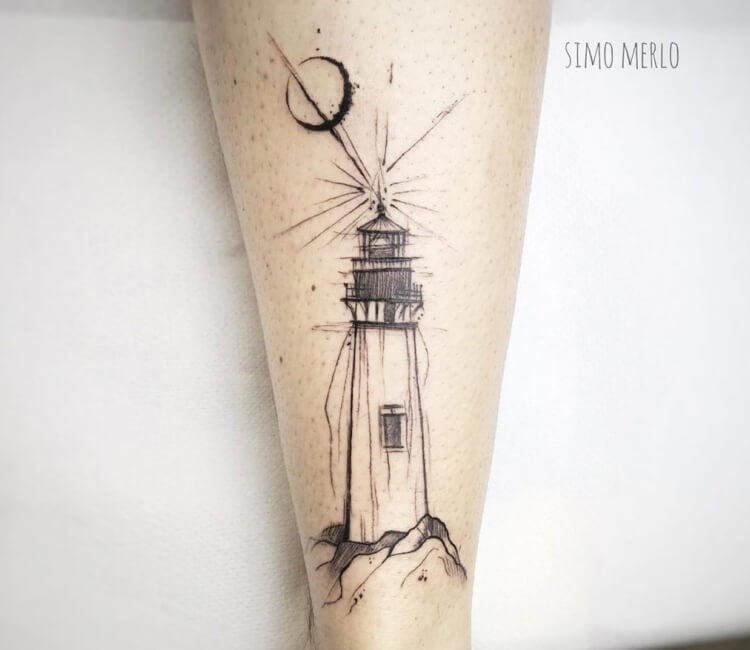The image showcases a freshly inked tattoo on what appears to be the back of a person's leg, potentially the calf. The grayscale tattoo prominently features a black-outlined lighthouse perched on a rocky or mountainous surface. The lighthouse emits beams of light from its top, indicating it is lit up. To the upper left of the lighthouse is a celestial body, likely a moon in an eclipsed or crescent-like phase, adding a mystical element to the scene. The tattoo is detailed, with careful shading to create depth, though unfinished as some parts may lack complete shading. A signature reading "Simo Merlo" is visible at the top right corner of the image. The person’s leg rests against a white background, providing a stark contrast that highlights the intricate artwork on the skin.